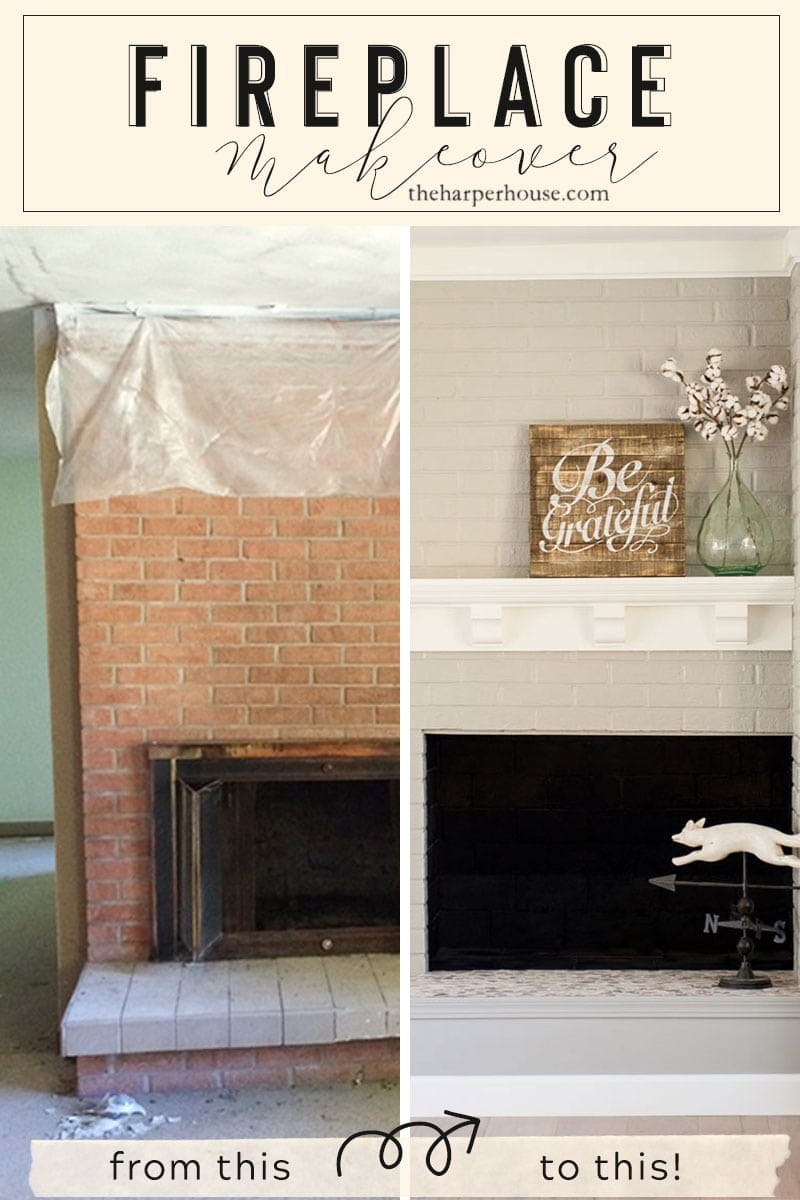The image illustrates a striking before-and-after transformation of a fireplace makeover. Against a beige background, the text "Fireplace Makeover by theharperhouse.com" is prominently displayed above the images. The narrative is further detailed with the words "from this to this" connected by a squiggly arrow between the before and after shots. On the left side, the fireplace is depicted in its original state: constructed from bright pinkish-orange bricks, adorned with foil hanging from the top, and some debris littered on the beige, untreated floor. On the right, the fireplace is shown post-makeover, boasting a sleek, modern appearance. The bricks are now painted a light gray, complemented by a pristine white mantle. Decorative touches include a wooden sign reading "Be Grateful," a clear vase containing white cotton flowers, and a wind compass ornament, adding both aesthetic and functional appeal. The revamped fireplace, possibly electric, transforms from a run-down feature into a stylish focal point, demonstrating a successful DIY renovation.